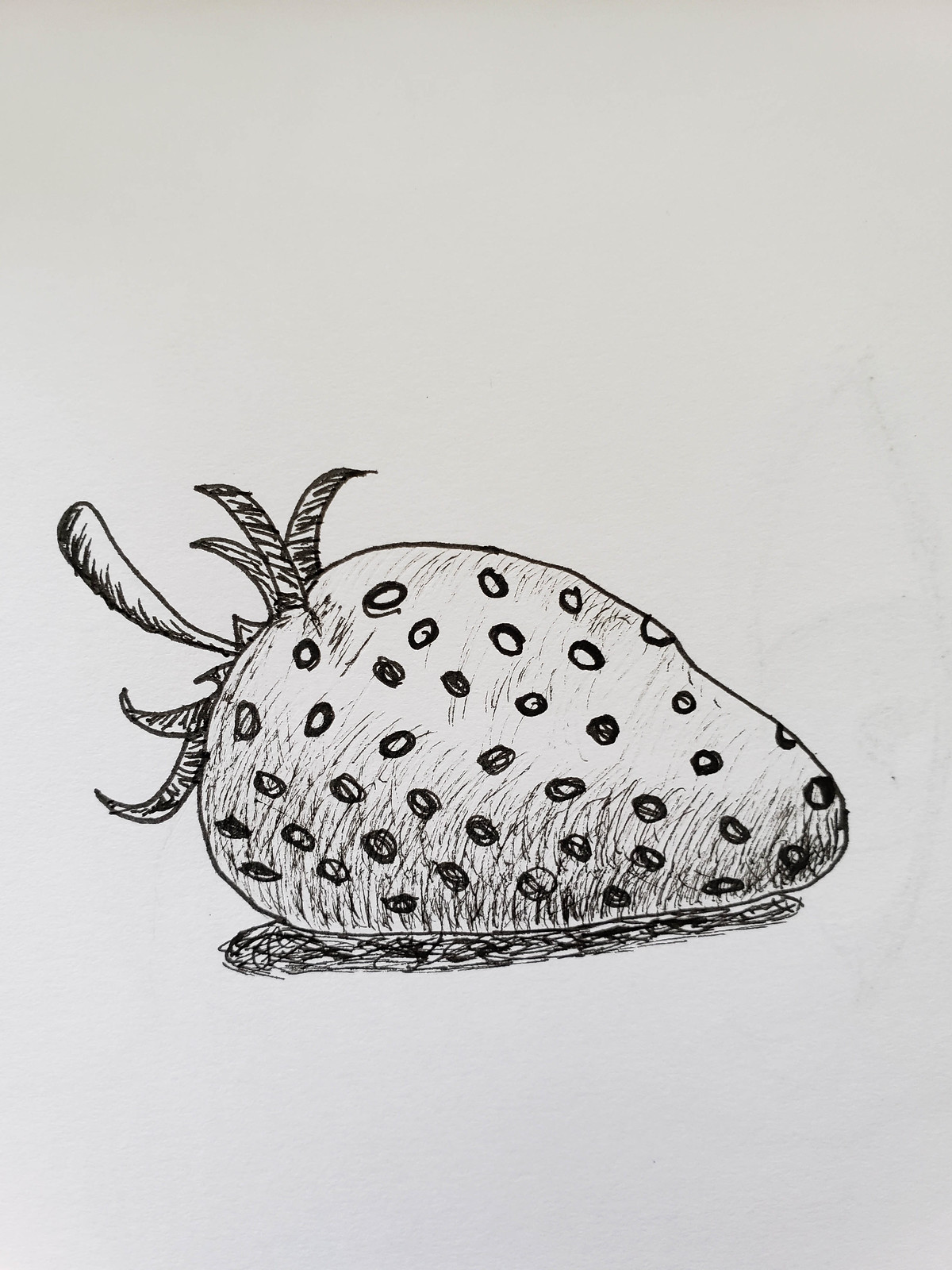This intricate black and white illustration features a highly detailed strawberry rendered in pen or pencil. The strawberry is positioned on its side with the stem extending to the left. The meticulous shading beneath the strawberry suggests it is casting a shadow, enhancing its three-dimensional appearance. At the top of the strawberry, the long stem is surrounded by a crown of seven leaves, five of which are elongated while the remaining two are shorter and more stubby. The absence of color emphasizes the texture and fine lines, capturing the essence of the fruit with remarkable precision.